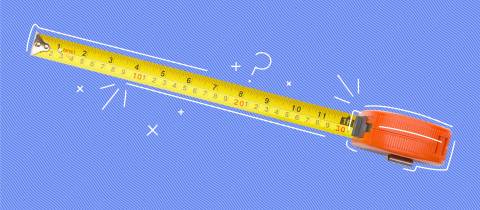This detailed color photograph showcases a tape measure arranged on a light blue background, viewed from a top-down perspective. The tape measure, featuring a yellow blade with black inch markings and an orange casing that exhibits a somewhat aged, brownish-tan appearance with hints of red, is extended to the 12-inch or one-foot mark. Elaborate white lines drawn around the tape measure emphasize its outline and tip. Surrounding the tape measure and drawn onto the background are various white illustrations, including multiple multiplication signs (one notably at the bottom), a plus sign, a question mark, an arrow pointing toward the 12-inch mark, and an additional arrow pointing up to the 4-inch mark. These added elements lend a whimsical or instructional feel to the otherwise utilitarian image of the 20-30 year old measuring tool.